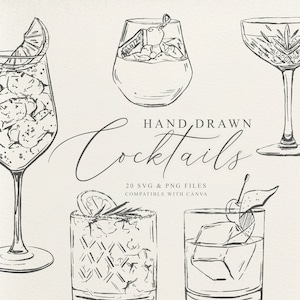The illustration features five distinct, hand-drawn cocktail glasses, rendered in black and white, set against an off-white background. Central to the image is the text "hand-drawn cocktails" displayed prominently, with "20 SVG and PNG files compatible with Canva" written below in smaller letters. Each glass is characterized by unique details: the largest glass on the left, likely a wine glass, showcases a half-cut lemon garnishing the top, with visible ice cubes inside. To its immediate right and slightly above, a smaller glass, possibly a highball or stemless wine glass, is half-filled, featuring a cherry in the center. In the upper right corner, a champagne or parfait glass stands out, while on the bottom left, a glass with a triangular pattern contains an orange slice and ice. Adjacent to it, a glass with a large ice cube and a garnish completes the arrangement. The overall color scheme is lightish blue, adding a cohesive backdrop to the detailed, pencil-drawn illustrations.